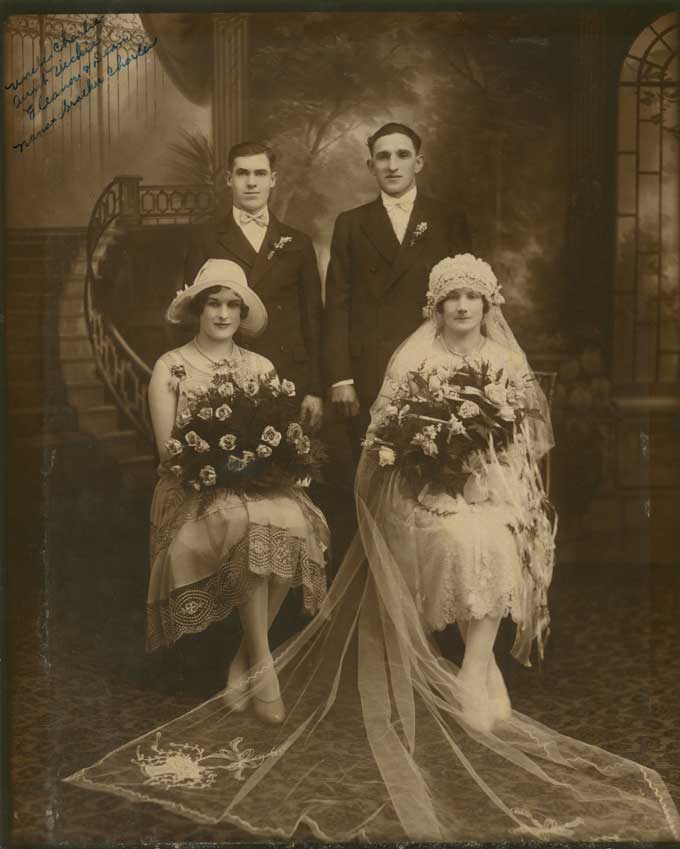The photograph is a sepia-toned, old-fashioned image, reminiscent of the early 20th century, showcasing a wedding scene with four individuals. The two women, sitting in ornate chairs, are adorned in elegant dresses and holding large bouquets of flowers. The woman on the right, presumably the bride, wears a flowing wedding dress complete with a long, expansive veil draped over the floor and a big shawl. The woman on the left, likely the bridesmaid or maid of honor, is dressed in a formal gown, accessorized with a hat, and also holds a bouquet. Behind them, standing in tuxedos, are two men, possibly the groom and best man, adding to the formal atmosphere of the scene. They are positioned in front of a grand staircase within a sophisticated, two-story building. The upper left corner of the image includes a cursive inscription, though it is difficult to decipher.